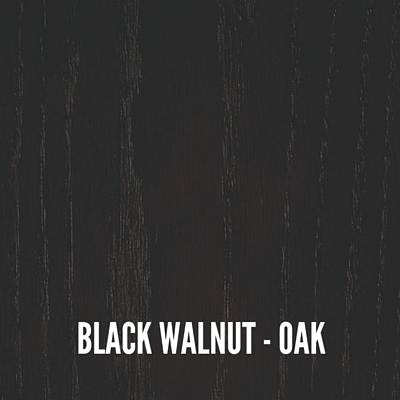The image depicts a square area shaded in deep black, featuring vertical striations that create a wood grain texture, resembling black-stained wood. This effect gives off a subtle mix of black and gray with notable lighter lines - approximately three or four on the left, one down the center, and another four on the right side, which together form a highlighted plank effect. The bottom edge of the image is marked with bold, all-uppercase white letters, centered, and reading "BLACK WALNUT - OAK" in a sans-serif font. This text suggests the image represents the color and grain pattern of black walnut oak wood.